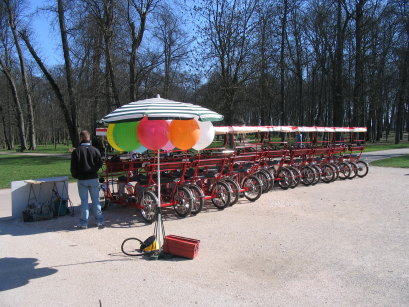The photograph captures a vibrant outdoor scene in a park on a sunny day. The image features a large paved central area framed by green grass and a backdrop of tall deciduous trees without leaves, suggesting it's taken in late autumn or early spring. Dominating the foreground is a line of red tandem bicycles, each with a white canopy and black tires, arranged diagonally across the pavement. Adjacent to the bicycles stands a large beach umbrella with blue and white stripes, anchored by a red box and holding a collection of brightly colored balloons in shades of yellow, green, pink, orange, blue, and white. A man in a black jacket and blue jeans stands with his back to the camera, facing the line of bicycles. The clear blue sky visible through the bare tree branches, along with the shadows cast by the umbrella, indicates it’s a bright, sunny day.